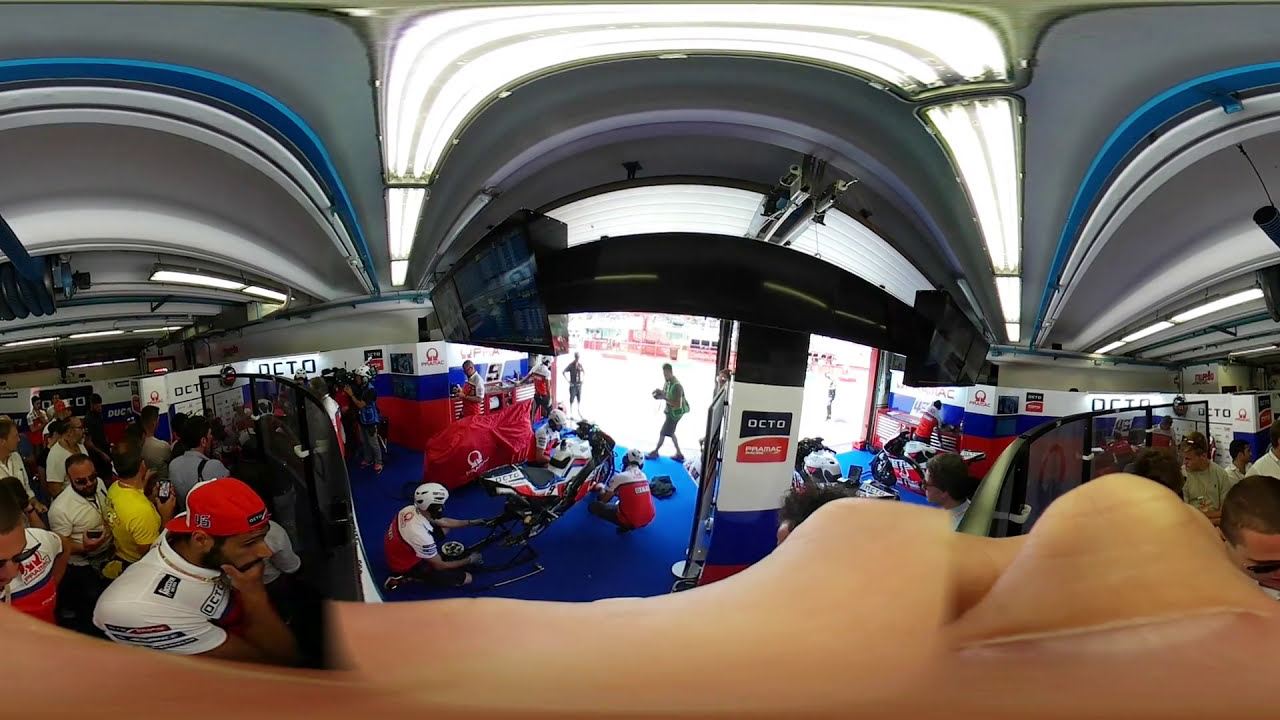The image captures the vibrant scene inside a bustling sports garage, designed for fans to observe their favorite racers work on bikes through a glass partition. The setting appears crowded, with people standing on a dark blue rug. In the foreground on the bottom left, a mechanic in a white helmet is crouched down, working on a motorbike missing its back wheel. He wears dark shorts and a distinct polo shirt that's white around the shoulders and red from the chest down. The bike he's fixing features a white, red, and blue color scheme with a black seat. Several individuals in uniforms identical to the mechanic's, along with caps or helmets, are scattered throughout the area, engaged in various tasks. The ceiling of the room alternates between blue and white, and a wide screen divides different sections of the room. The image is taken from a perspective that includes flesh-colored fingers at the bottom, giving the impression of a panoramic view from a high vantage point, possibly atop a shelf.